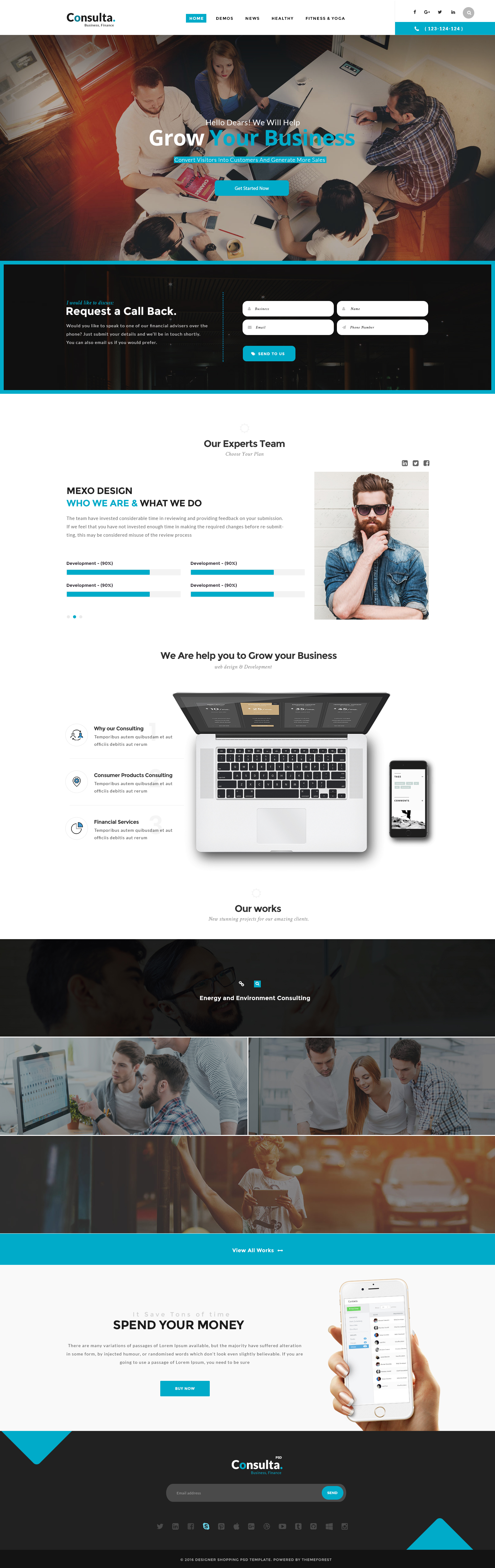In this screenshot, we see an intricately designed landing page aimed at helping businesses grow. At the top, the page prominently features the tagline "Grow Your Business" in bold text. Below this, there is an opt-in form labeled "Request a Callback" where users can input their name, phone number, and email address.

The center of the page showcases a series of visuals: a picture of a gentleman, a computer, and a tablet. Accompanying these images is a section introducing "Our Expert Teams" with the header "Mexo Design." Though the accompanying text description is too small to read, it’s meant to provide further details on the team and their services. The repeated word "development" underscores their focus on business growth through various developmental strategies.

Further down, there is a statement: "We are here to help you grow your business." This is followed by a picture of a laptop. Another section asks, "Why our consulting?" and features several icons representing different fields of expertise like consumer products consulting, financial services, and energy and environment consulting.

The landing page's color scheme prominently uses turquoise and black, contributing to a professional yet approachable aesthetic. Lastly, the page includes prompts such as "Spend Your Money" and "Consulta," perhaps encouraging users to explore further consultation services.

In summary, the landing page offers a comprehensive overview of Mexo Design's consulting services, supported by visuals and an easy-to-navigate interface focused on engaging and assisting potential clients.